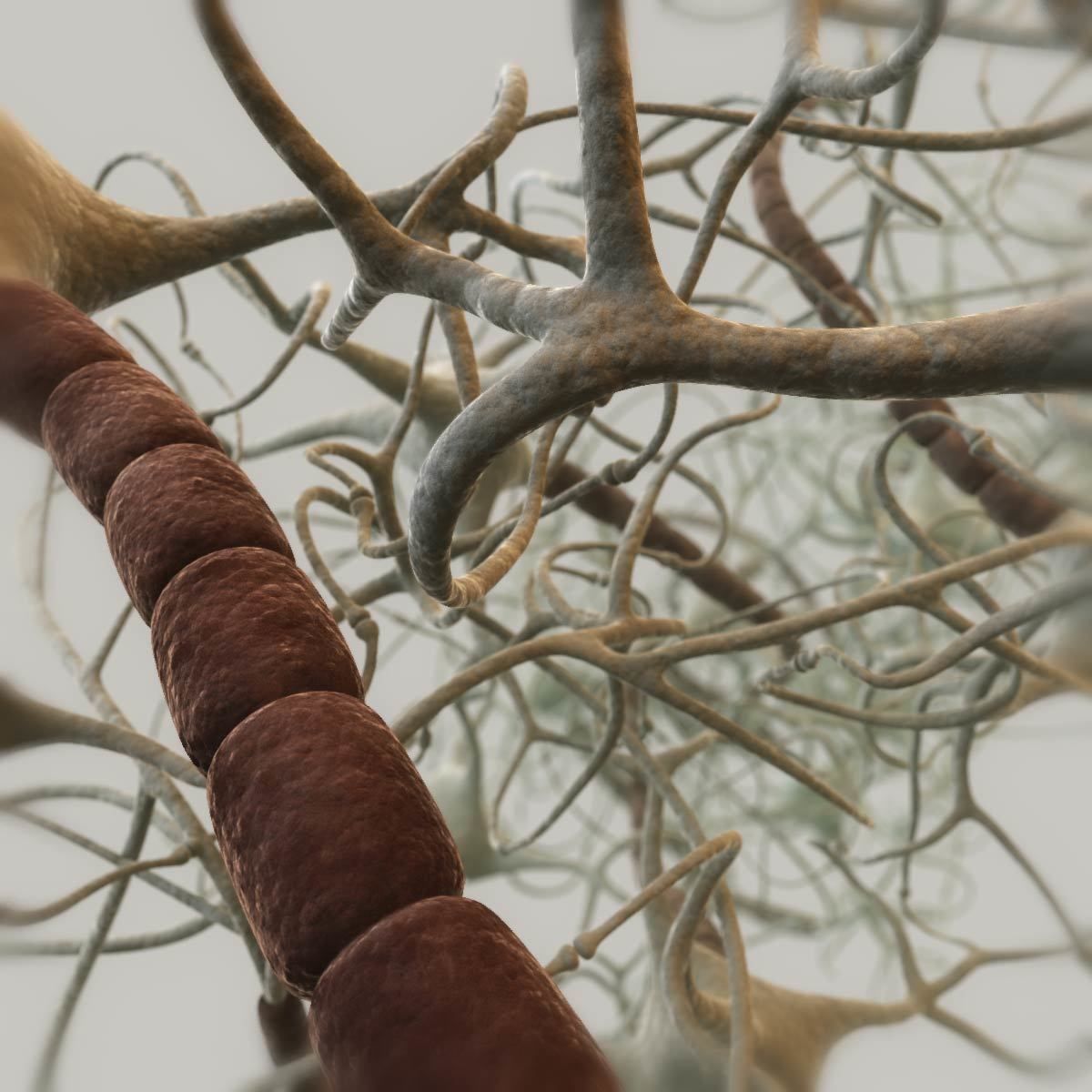This detailed and intriguing image presents a multi-colored, perfectly rectangular scene without borders. The background is a simple gray, creating a stark contrast with the intricate foreground. Dominating the image is a complex network of twisting, interwoven structures that resemble bare tree branches or biological tentacles. With shades primarily in brown, dark beige, and some striking red and burgundy segments, these structures evoke the appearance of neurons or microscopic connections within a body. Towards the left side, there's a peculiar stack of red, marshmallow-like shapes, almost reminiscent of deer antlers. The overall impression is that of a mesmerizing, possibly computer-generated rendering of a biological or microscopic phenomenon, free-floating in an otherwise empty space.